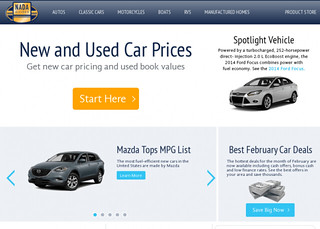The website features a sleek design with a navy blue banner at the top, complemented by darker blue lines at both the top and bottom edges. An eye-catching gold-bordered icon labeled "CATA" (K-A-D-A) is positioned prominently at the top. The navigation bar includes options for Autos, Classic Cars, Motorcycles, Boats, RVs, Manufactured Homes, Product, and Store.

Beneath the banner, the website boasts a white background showcasing key information in navy print: "New and Used Car Prices" with subtext reading "Get new car pricing and used book values." A prominent yellow-orange button marked "Start Here" in white print, accompanied by a rightward arrow, invites user interaction.

Adjacent to this section, "Spotlight Vehicle" introduces a featured car, the "2018 Ford Taurus," highlighted in blue text. 

The lower section of the site transitions to a gray background divided into two segments: a rectangle and a square. The rectangular section, labeled "Mazda Top MPG List," features an image of a car flanked by navigational arrows on either side. The square segment highlights "Best February Car Deals," adorned with an image of a pile of money and a blue clickable tab.